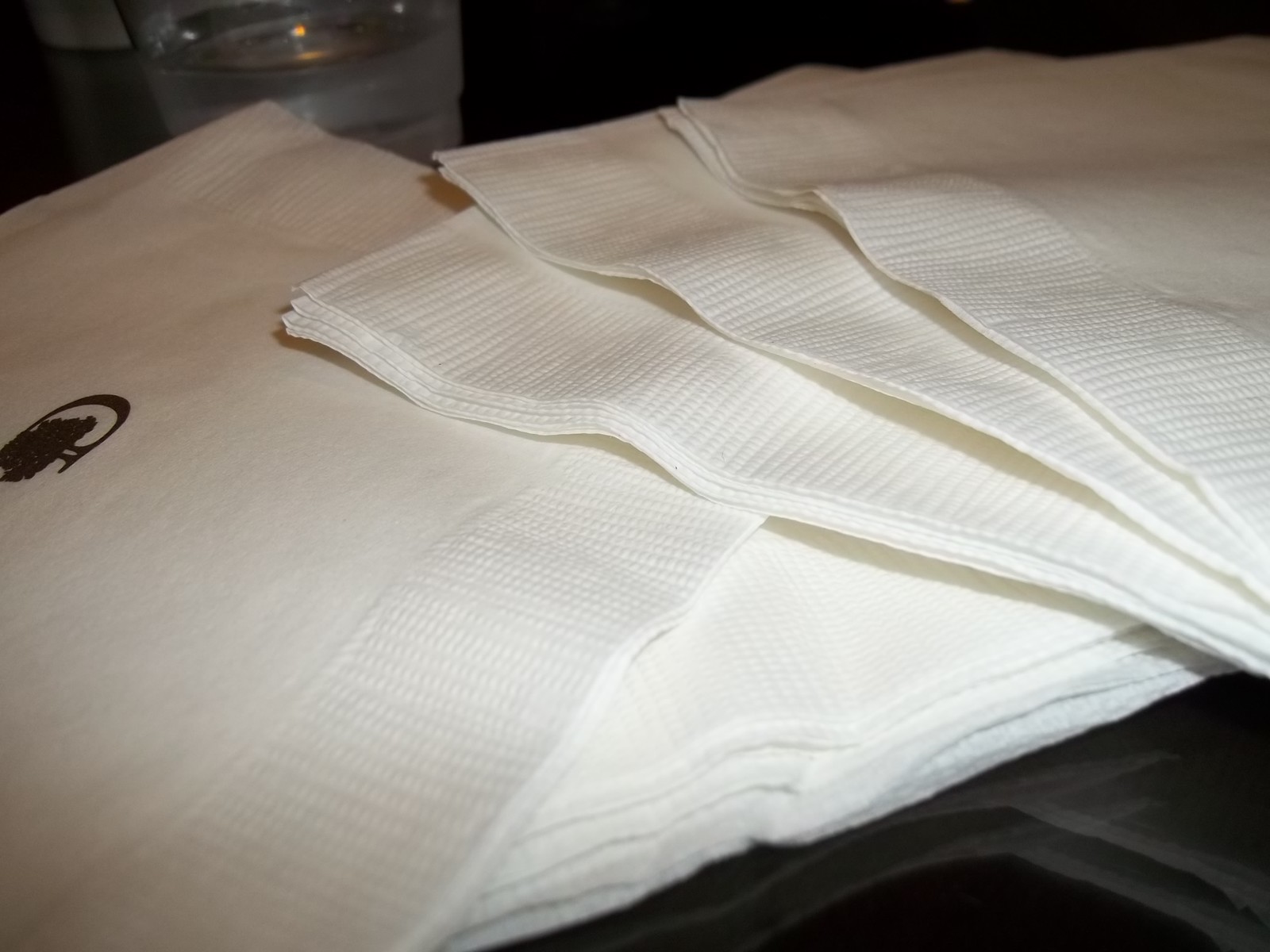The photograph captures a close-up of a slightly disheveled stack of high-quality, branded white napkins on a black, mirror-finished surface, possibly a kitchen countertop or a bar table. The surface is reflected due to its glossy finish, and a glass of water can be seen in the background, suggesting an establishment setting such as a restaurant or bar. Prominent on one of the napkins is a black logo featuring a letter D intertwined with a tree design, likely representing the establishment’s brand. The napkins are arranged with some neat stacks to the left, though one napkin is notably slanted at a 40-degree angle. The lighting, coming from the right side of the image, casts subtle highlights, reinforcing the professional quality of the napkins and the setting.